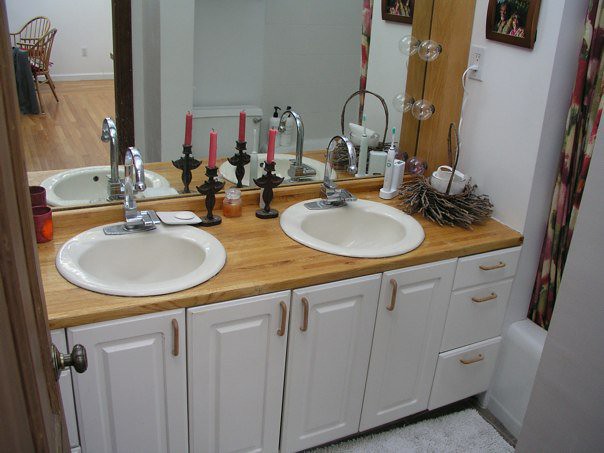This image depicts a meticulously organized bathroom, likely designed for a couple or a partnership, evident by the presence of dual amenities. Dominating the scene are two circular sinks, positioned symmetrically on a wooden countertop that harmonizes with the frame of the large mirror mounted above. Each sink is complemented by a pink candlestick of identical size, adding a touch of elegance and romance to the space.

To the left of the first sink, there is a red cup, along with a soap dish holding a bar of soap. The right sink features an electric toothbrush settled in its holder. Adjacent to this toothbrush is a basket resembling a nest, containing an enigmatic bucket. 

The mirror reflects additional furnishings, revealing two chairs and a portion of a table, hinting at an adjoining room. To the right of the second sink, there is a picture frame, and partially visible is a bathtub with its corresponding curtain. The pristine white cabinets below contrast beautifully with the rich wood of the countertop, creating a cohesive and inviting atmosphere.